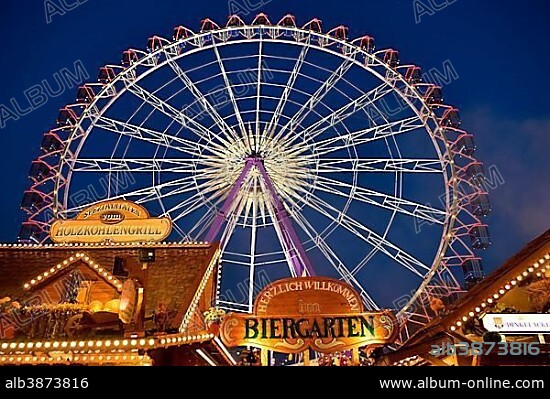The image is a business advertisement with a striking dark blue background and white text. Dominating the scene is a large Ferris wheel with purple and white framework, illuminated with golden lights that give it a bright, inviting appearance. The Ferris wheel is positioned behind two illuminated buildings, whose rooftops are adorned with small circular light bulbs. One building on the left displays a sign reading "HOLZKOHLENGRILL," while another centrally placed sign reads "HERZLICH WILLKOMMEN IM BIERGARTEN" on a gold background. Adding to the detail, a small alphanumeric code, "ALB3873816," is seen on the right corner just above a black border running along the bottom. This black border also features the website "www.album-online.com" on the right and the same alphanumeric code "ALB3873816" on the left. The overall scene, with German text and the festive lighting, suggests that the image was likely taken in Germany.